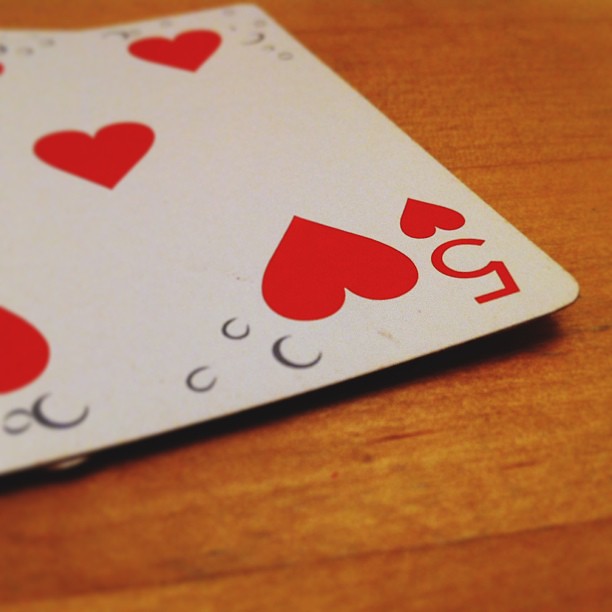The image depicts a playing card, specifically the five of hearts, positioned upside down on a wooden table. The card lies heart-symbol side up, revealing distinctive details of its surroundings. The wooden table surface showcases intricate wood grain patterns, with varying shades from lighter tannish-yellow hues to deeper red tones. Scattered over the card are small water-like droplets concentrated more towards the middle and edges rather than the numbered areas. These could potentially be black C-shaped imprints, although it's challenging to determine their exact nature. The playing card does not rest flat but appears slightly elevated, suggesting something underneath it that creates a minor lift.